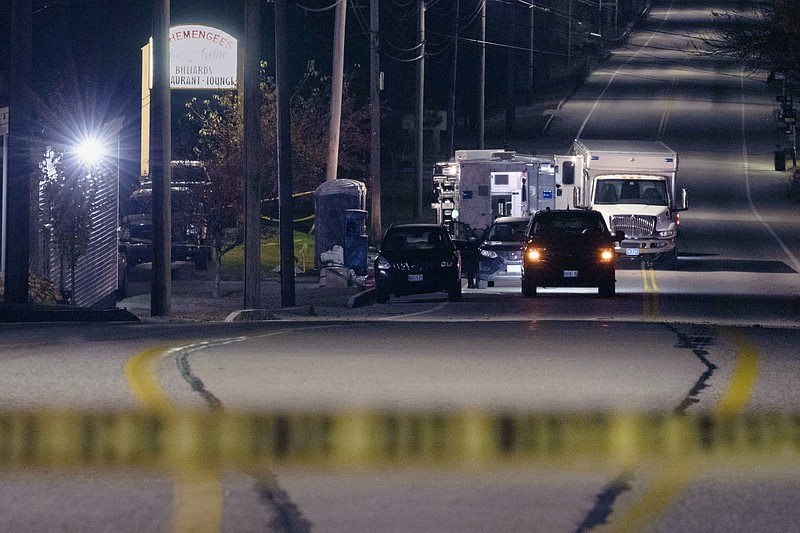The image captures a nighttime scene on a slightly hilly, paved street outside a billiard lounge named "Heminges Billiards Restaurant Lounge." The scene is lit by street lamps on utility poles that line the left side of the road. The main focal point is a cluster of vehicles suggesting a potential accident. In the foreground, an out-of-focus police barrier or caution tape runs across the image. 

At the front of this cluster, two black SUVs face the viewer, with the one on the left having its headlights on. Immediately behind these SUVs, a passenger car has its passenger door open, revealing a person's legs and feet. Further back, two white box trucks are aligned, both with their doors open and unmarked, while to their right stands a white ambulance with its rear doors open and blue lights visible at the back, hinting at emergency response activity.

To the left of the scene, there's a porta potty and a trash can positioned on the sidewalk. The left side of the image also reveals the billiard lounge, identifiable by its vinyl siding and illuminated sign. Additional details include tree branches and grassy areas visible around the scene, underlining the suburban setting of this nighttime occurrence.